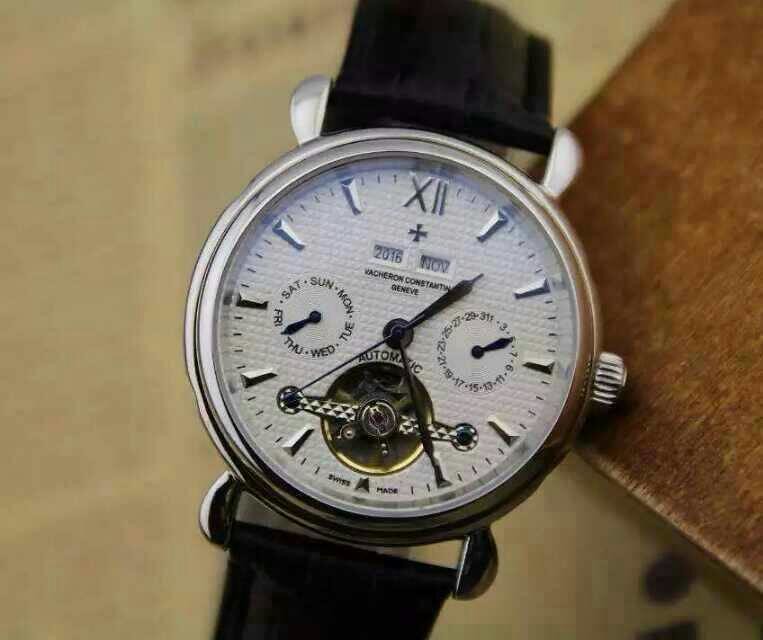This image showcases a meticulously designed wristwatch, prominently featuring the elegant face of the timepiece, slightly tilted to the right. The watch sports a sleek black band, paired with a polished silver bezel that frames the watch face. The pristine white dial contrasts beautifully against the black and silver accents.

At the top of the dial, a sophisticated silver Roman numeral "12" marks the hour, while thick silver indices denote the other hours and finer lines mark the minutes. Dominating the center is an intricate gold circle, featuring a crossbeam design that reveals the mesmerizing gears within—a delightful preview of the watch's automatic movement, which is proudly labeled above this gold section.

The watch face is further adorned with the prestigious name "Vacheron Constantin Geneve," highlighting the brand's esteemed heritage. Below the brand name, a series of small rectangles display "November 2016," with a central plus sign among them, indicating perhaps a special edition or commemorative detail.

On the right side of the watch face, the textured crown, or winder, is distinctly visible and adds a functional charm to the timepiece as it gently leans against a rustic wooden box—providing a warm, blurred backdrop that enhances the watch's refined presentation. Additional features include a sub-dial to the left of center that indicates the date, and another sub-dial to the right displaying a sequence of higher numbers, likely related to a secondary time-telling function.

Overall, this watch is exquisitely displayed, ready to captivate potential buyers or horology enthusiasts with its blend of luxury, craftsmanship, and detailed artistry.